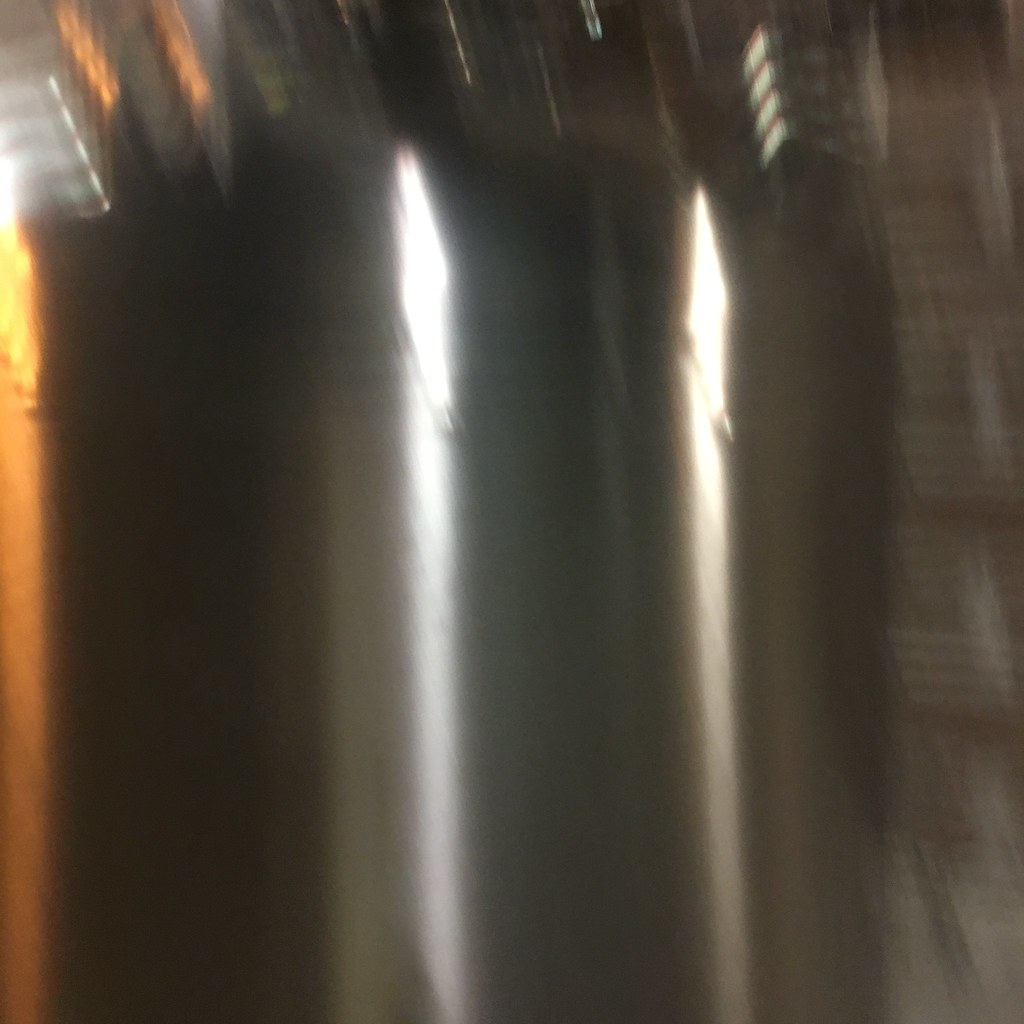This grainy and poorly lit photograph features a metallic, brushed silver cylinder positioned at an angle that creates a diagonal blur. The cylinder, likely made of metal, has two distinct beams of reflection upon its surface. Several protrusions emerge from a presumed lid at the top of this cylindrical object, adding to its complexity. In terms of lighting, the image has a soft, light-colored illumination in the foreground. Additionally, a yellow backlight is visible to the left of the cylinder, casting a faint glow. To the right, there appears to be a brick wall, partially visible and contributing to the overall setting.